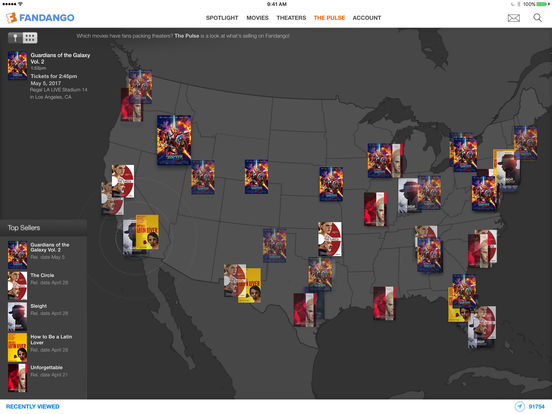This detailed caption should accurately convey all the elements described in the screenshot:

"This screenshot from Fandango features several key elements. At the top, in all-capital blue letters, 'FANDANGO' is displayed, with a white 'F' outlined and accented in orange to the left of the word. Centered on the header, the time '9:41 AM' is shown alongside menu options including 'Spotlight,' 'Movies,' 'Theaters,' 'The Pulse,' which is currently selected, and 'Account.' On the far right are email and search icons. 

The main section displays a gray map of the United States outlined in black, overlaid with numerous movie posters indicating what films are playing in different regions. At the top left of this map, details for a specific movie booking are shown: 'Guardians of the Galaxy Vol. 2' for 2:45 PM on May 5, 2017, at 'Regal LA Live Stadium 14' in Los Angeles, CA.

At the bottom left, a list of top sources is displayed, featuring movie titles such as 'Guardians of the Galaxy Vol. 2,' 'The Circle,' 'Sleight (spelled S-L-E-I-G-H-T),' 'How to Be a Latin Lover,' and 'Unforgettable.'"